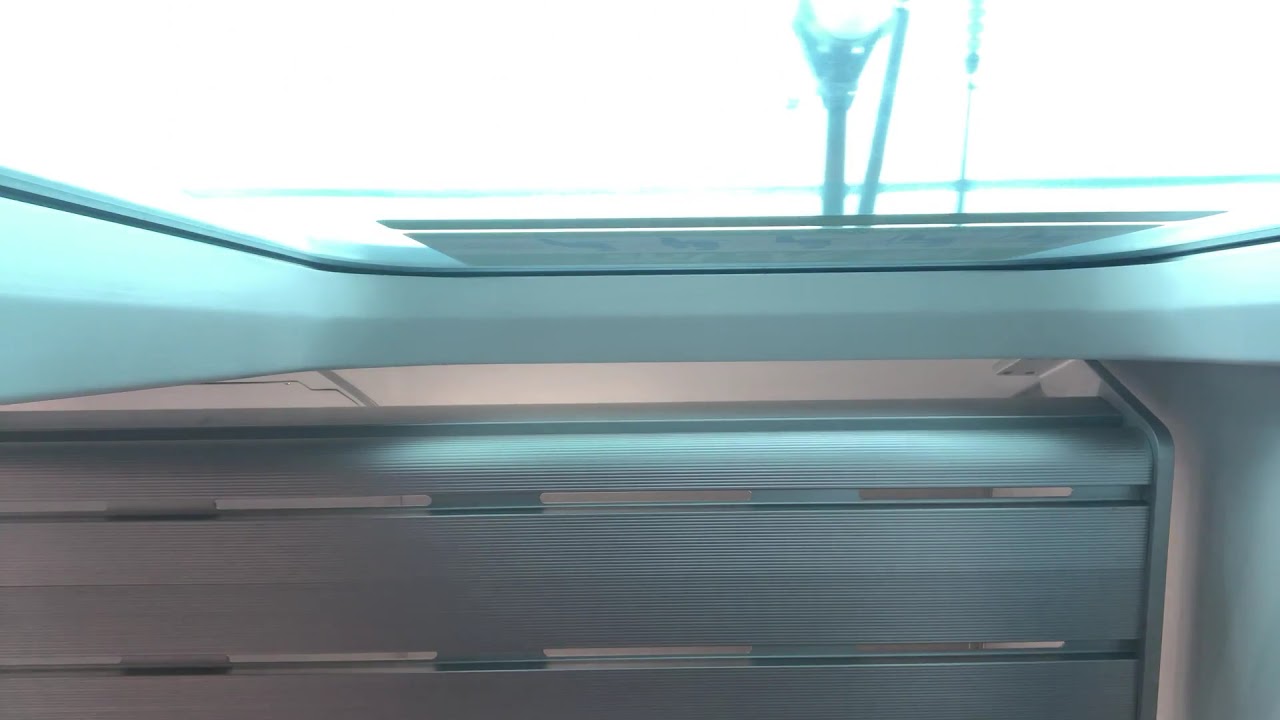The image displays a highly zoomed-in, somewhat challenging view inside a confined space, likely a vehicle such as a plane, bus, or train. Dominating the top portion of the image is a blindingly bright skylight or window bordered by white plastic, suggesting PVC material. The window appears to have an indistinguishable sticker on it, and outside, tall, thin poles are visible. The bottom half of the image features gray metallic sections, likely resembling a closed steel grate, indicative of an overhead baggage storage area. The bright light from the window partially obscures some details, casting a hazy glow across the scene. The image below the window is further characterized by structured tiers and indentations, hinting at the organized compartments found in public transport interiors.